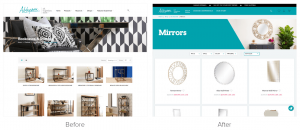This image appears to be a collage from a home decor retailer's website, though the specific retailer is not identifiable due to the small image size. On the left side, it showcases various table options available for purchase, likely catering to different styles and preferences. The tables are presented under the heading "Before." Adjacent to this section is another displaying an array of mirrors, both circular and rectangular, accompanied by the heading "After." The collage suggests the idea of enhancing a table setup by adding a mirror above it. Despite the cohesive color scheme connecting both sections, the screenshots seem to originate from different webpages, possibly even different websites. The overall cohesiveness is undermined by the disparity in layout and detail resolution. Pricing and additional category information are not visible due to the small image and text size, making it difficult to extract further specifics.